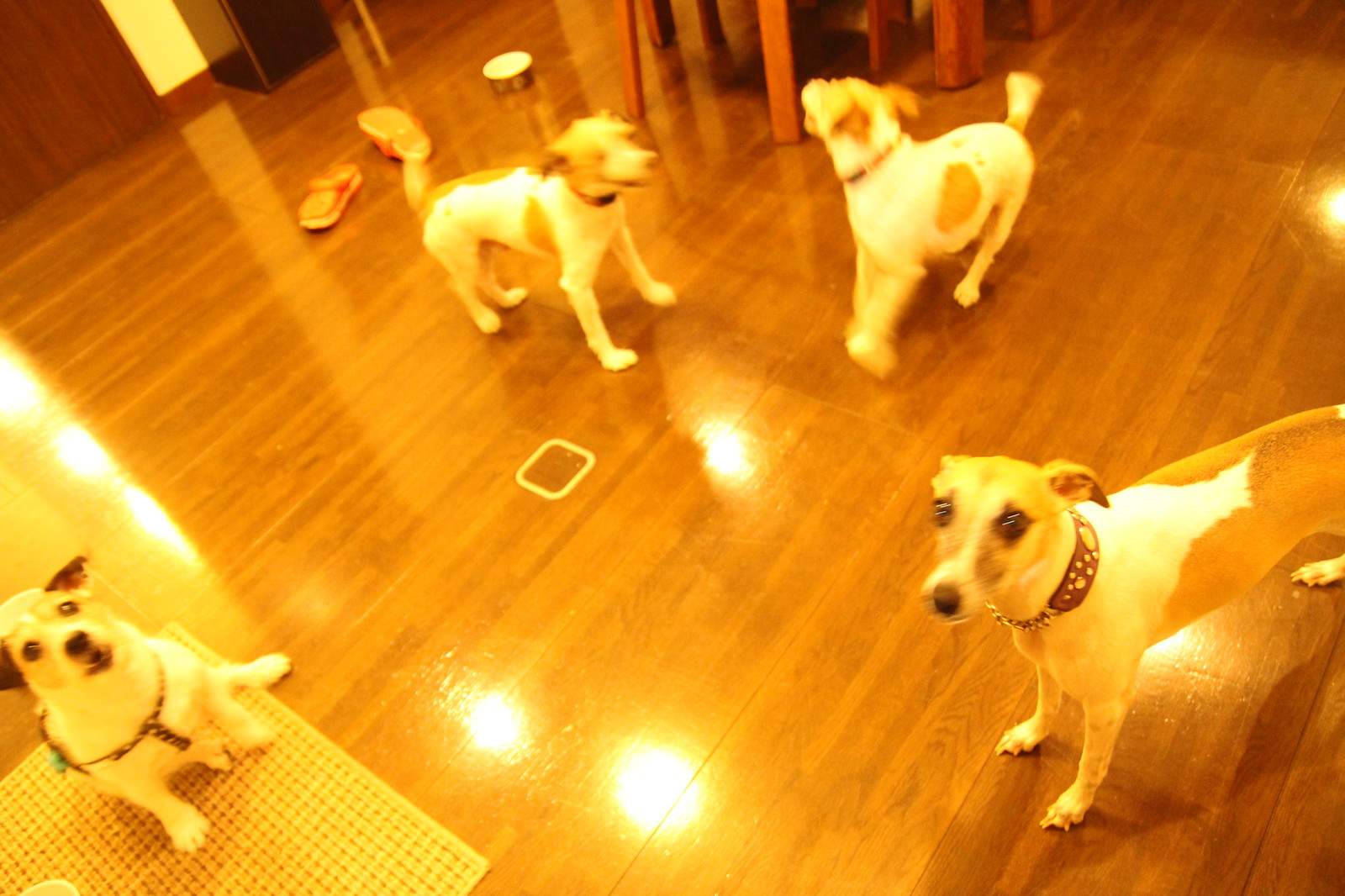In this detailed image, four small to medium-sized dogs are featured on a shiny, hardwood floor that reflects the overhead lighting, creating noticeable glare. The two dogs in the foreground are staring directly into the camera, their brown and white coats suggesting a terrier breed with perhaps some corgi influence. Both have brown leather and chain collars, with the one on the left also wearing a brown harness. In the background, two more dogs are engaged in playful activity, appearing blurred in motion; one seems to be barking. To the left side of the image, a dog sits on a mat near a partially visible dog food bowl, while scattered objects such as a pair of slippers and some chair legs can be seen, adding to the casual, lived-in feel of the scene. There are additional slippers in the upper left corner, enhancing the impression of a homey environment. The overall composition captures a candid moment of domestic life, with the dogs' inquisitive and lively expressions drawing immediate attention.